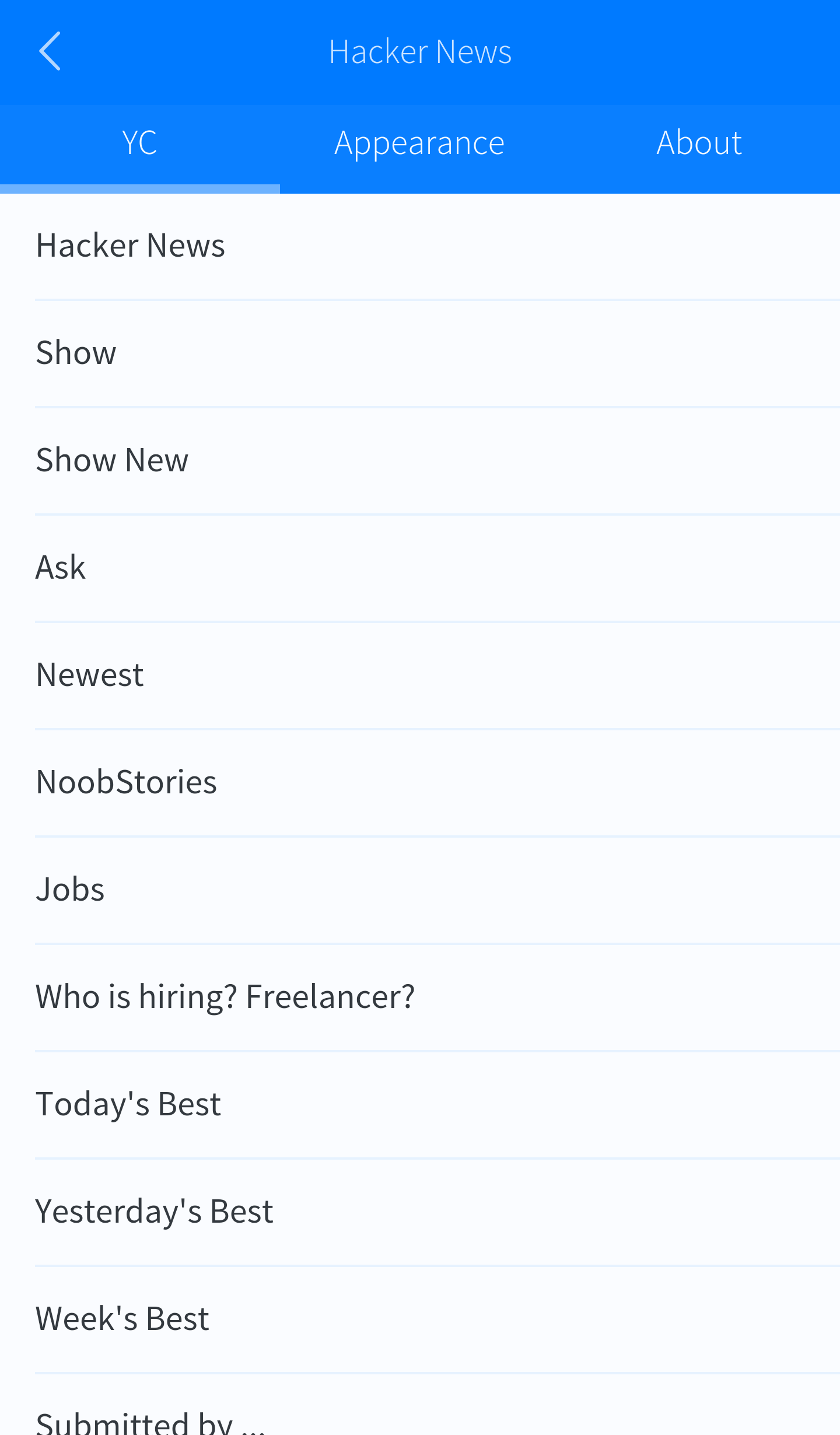The image is a tall rectangular snapshot from an online source, prominently featuring the website Hacker News. At the top, a royal blue banner spans the width of the image. In the center of this banner, "Hacker News" is written in light blue lettering. Below the "Hacker News" title, the word "Appearance" appears in a slightly lighter shade of blue. Flanking the word "Appearance," the term "About" is situated to the right, and "YC" (short for Y Combinator) is placed to the left, both in capital letters.

In the upper left corner of the banner, there is a left-pointing arrow icon. The section below the blue banner features a white background, designed to resemble faintly lined notebook paper, with horizontal lines demarcating vertical sections.

Aligned along the left-hand side under the blue banner are several dark gray text items, each on a separate line. The sequence is as follows:
1. Hacker News
2. Show
3. Show New
4. Ask
5. Newest
6. Noob Stories
7. Jobs
8. Who is Hiring?
9. Freelancer? (This is all on one line following "Jobs")

Continuing down the list:
10. Today's Best
11. Yesterday's Best
12. Week's Best
13. Submitted By

Altogether, there are 12 distinct lines of text, each labeled in dark gray, providing various navigational or content-related options within the Hacker News site.